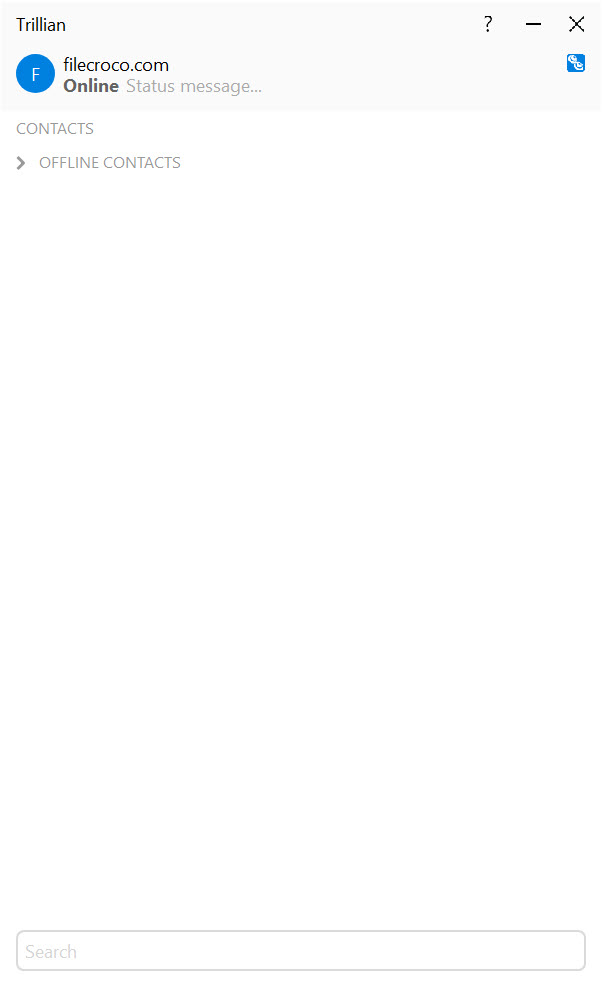The image depicts what appears to be either a phone screen or a website with a minimalist design dominated by white space and sparse details. At the top of the screen is a light gray box containing the word "Trillion" in dark gray text. Positioned below "Trillion" is a blue circle with the letter "F" inside it, and next to this is the text "File" followed by the URL "C-R-O-C-O dot com." Below this segment, in bold black text, is the word "online," with a subtler gray text below it reading "status message." To the right of these elements are a question mark, a dash, and an "X" symbol, each accompanied by a blue square logo underneath the "X." 

Beneath this, a white box displays the word "contacts" in gray text. Further down is a right-pointing arrow labeled "offline contacts." Between these sections is a search bar placed against an ample amount of empty white space, contributing to the minimalistic aesthetic of the interface. At the very bottom, there is another light gray search bar with the word "search" inside it, set within a long horizontal rectangular field, devoid of any additional elements.